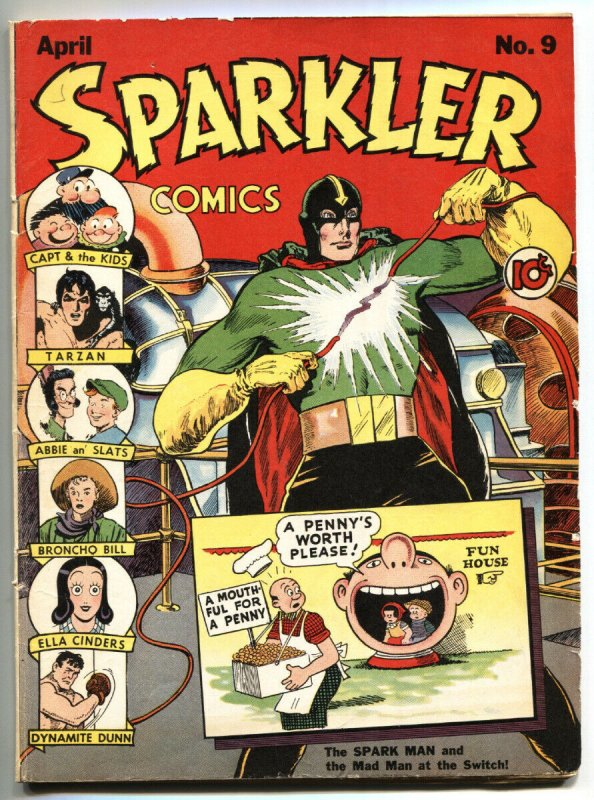The cover of the comic book titled "Sparkler Comics," issue number 9 from April, features a striking red background with bold yellow jagged letters proclaiming the title. Dominating the scene is a superhero in a dynamic pose at the center, gripping two red wires producing a vivid white spark. This hero is outfitted in a green bodysuit with yellow sleeves, black pants, a yellow belt with an orange section, and a distinctive black helmet mask adorned with a yellow arrow descending from the top to his eyes. Surrounding the superhero, the left side lists characters such as Captain and the Kids, Tarzan, Abby and Slats, Bronco Bill, Ella Cinders, and Dynamite Dunn. On the right side, a circular label indicates the price of 10 cents, and nearby, there's a promotional placard with the playful message: "A Penny's Worth Please, Fun House, A Mouthful for a Penny." In the bottom right corner, an additional cartoon illustration is visible, adding to the enticing preview of the comic's diverse content.